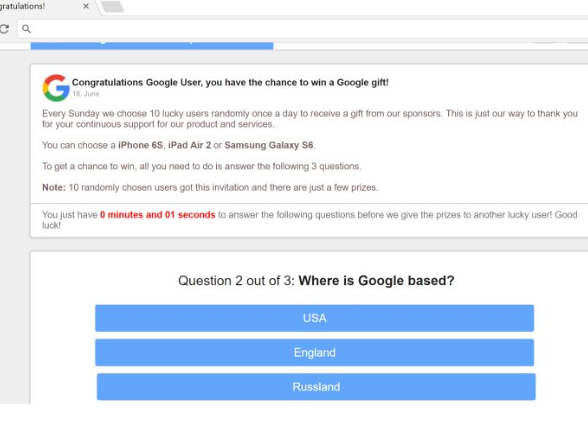The image is a screenshot of a suspicious message resembling a trivia quiz. At the top, it reads "Congratulations Google User! You have the chance to win a Google gift." The message states that every Sunday, ten random users are selected to receive a gift from sponsors, as a token of appreciation for their continuous support of Google products and services. The possible gifts are an iPhone 6s, an iPad Air 2, or a Samsung Galaxy S6. To be eligible for the prize draw, recipients are instructed to answer three questions. The screenshot highlights "Question 2 out of 3: Where is Google based?" with the multiple-choice options being USA, England, or Russian land. The message also mentions a time constraint, indicating that only one second is left to answer before the opportunity is given to another user.